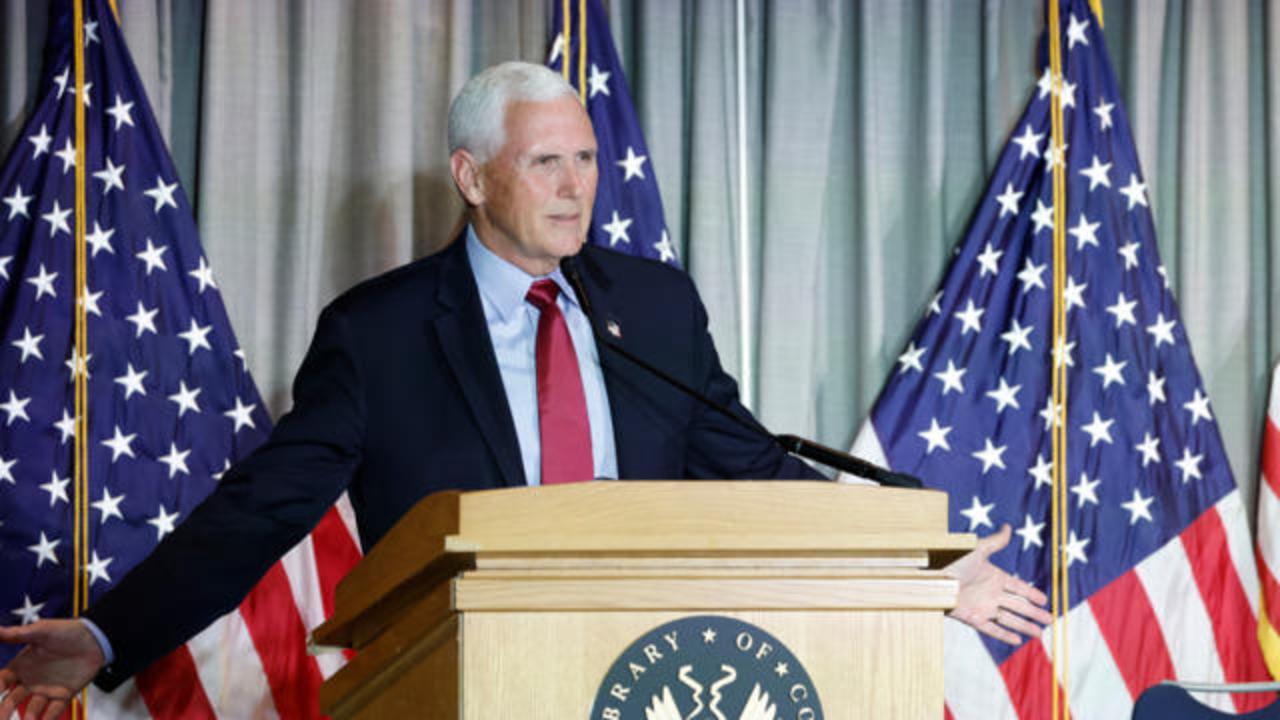This image captures former Vice President Mike Pence standing behind a wooden podium with a black logo that reads "Library of Congress." He is positioned in front of a backdrop of gray curtains stretching from the top to the bottom of the frame. Behind him are three U.S. flags on flagpoles, displaying red stripes and white stars against a blue field. Pence, dressed in a dark black suit, a light blue button-down dress shirt, and a bright red tie, stands with his white-haired head held high and arms outstretched to his sides. His expression, though neutral, suggests a moment of contemplation or mild agitation as he looks forward. The setting appears to be an auditorium where he is likely delivering a speech.